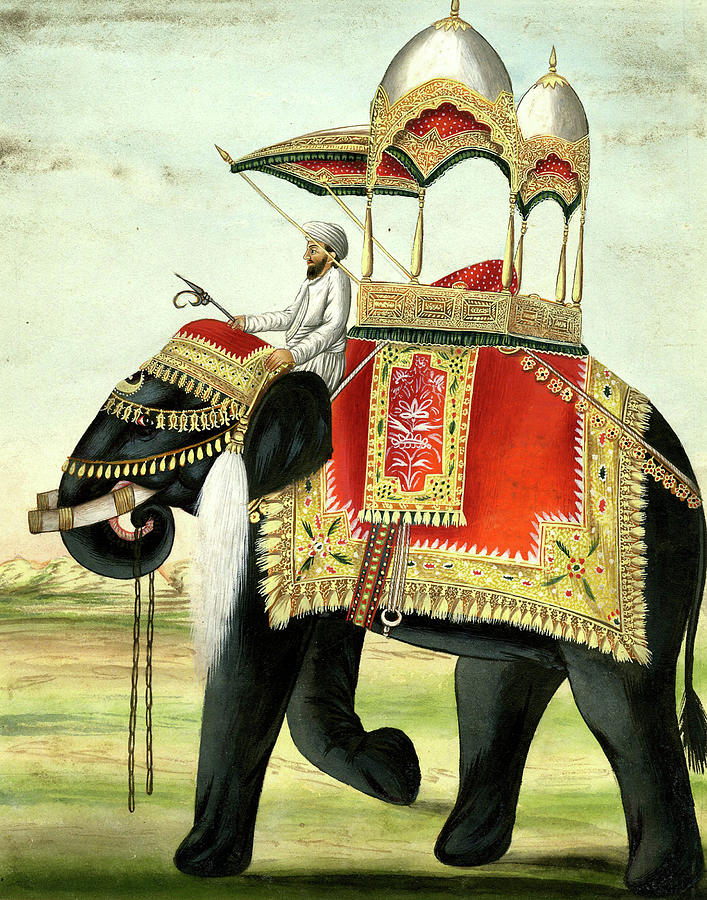An intricately detailed painting showcases an imposing black elephant adorned with elaborate gold embellishments on its head and around its trunk. The majestic creature dons a vibrant red blanket that drapes across its back, partially covered by gold detailing, possibly symbolizing a harness. The elephant's trunk curls upward, and its right front leg is bent, displaying a sense of movement. A man clad in white garments and a matching turban sits atop the elephant near its neck, riding in a seat that resembles a small gazebo. He holds what appears to be a poker. Despite the background being somewhat minimalistic and unfinished, the artwork exudes a regal, almost royal ambiance reminiscent of traditional Indian royalty. The elephant occupies a significant portion of the canvas, underlining its grandeur and dominant presence in the composition.